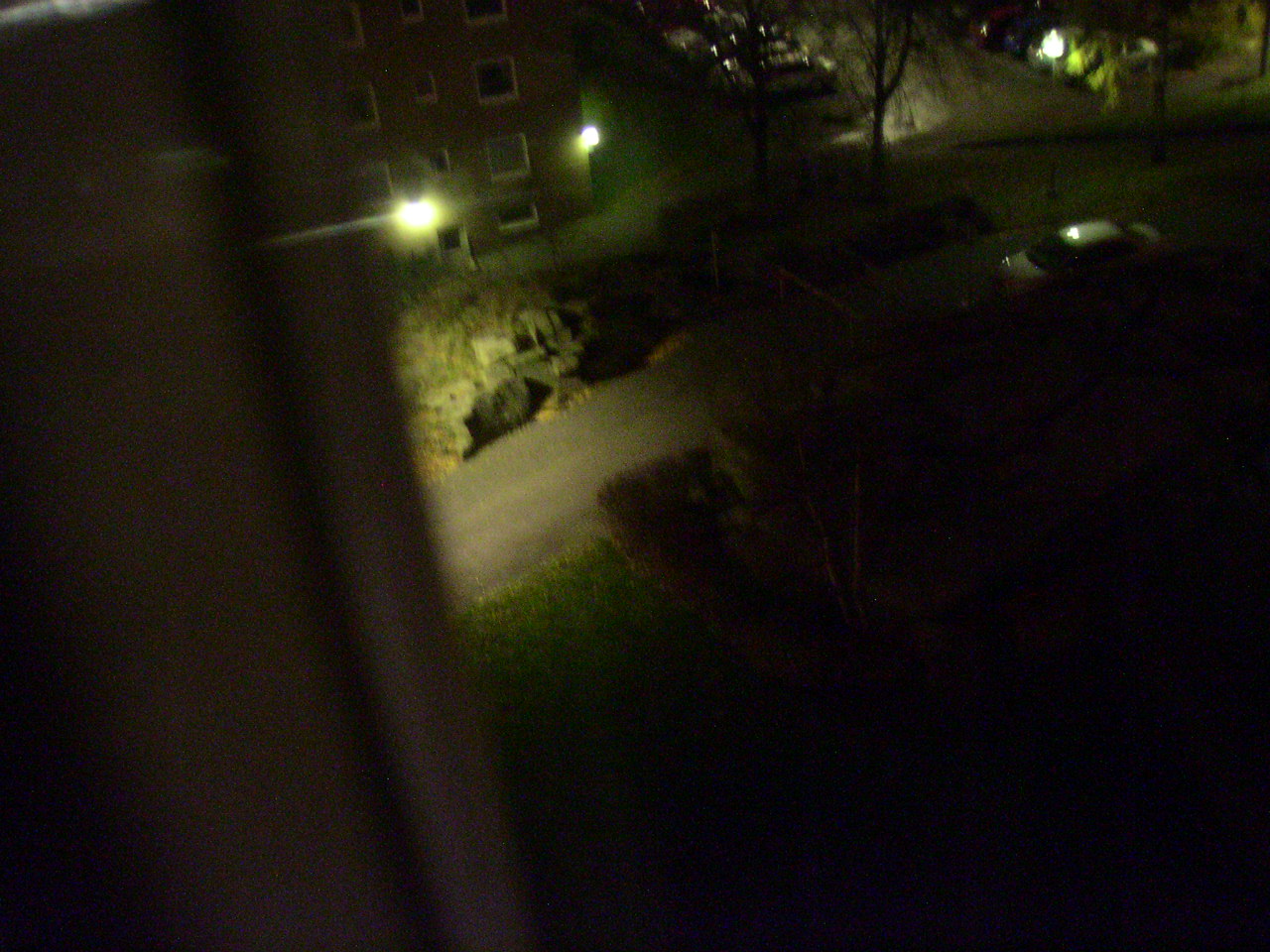A nighttime photograph taken from a higher-story window captures a view of the street below and a multi-story apartment building across the way. The windowsill and its edge are visible in the foreground, framing the shot. The illuminated apartment building features numerous windows, each offering a glimpse into the lives inside. Bright floodlights on either side of the building cast a stark glow, highlighting the grassy yards and parked cars lining the street. The scene evokes a sense of urban life, with the mixture of artificial light and darkness creating a contrast that draws attention to the architectural elements and the serene yet bustling ambiance of the neighborhood.